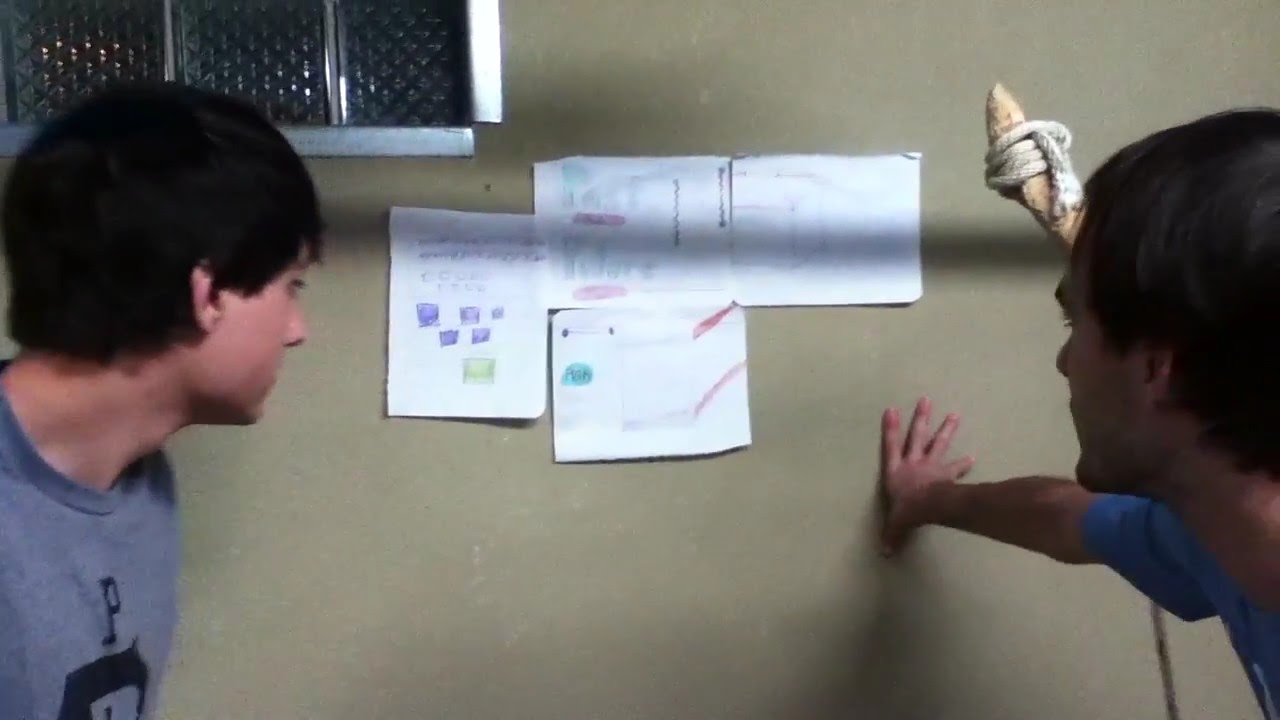The photograph captures a moment where two men, both with short dark brown hair, are intently examining four pieces of A4 paper taped to a light gray wall in what appears to be an indoor setting, potentially a basement. Both men are visible from the profile, with the man on the left wearing a gray T-shirt, and the man on the right in a blue T-shirt, his right hand reaching out and touching the wall. The papers, placed centrally on the wall, feature various colored markings, including purple squares, a lime green box, a teal oval, and reddish scrawls, all of which remain indistinct due to the distance and slight blur of the image. Above them, in the upper left corner, three square windows with thick, opaque glass framed in white can be seen. A wooden pole wrapped with white rope stands close to the wall behind them, adding to the detailed environment these men are engrossed in investigating.